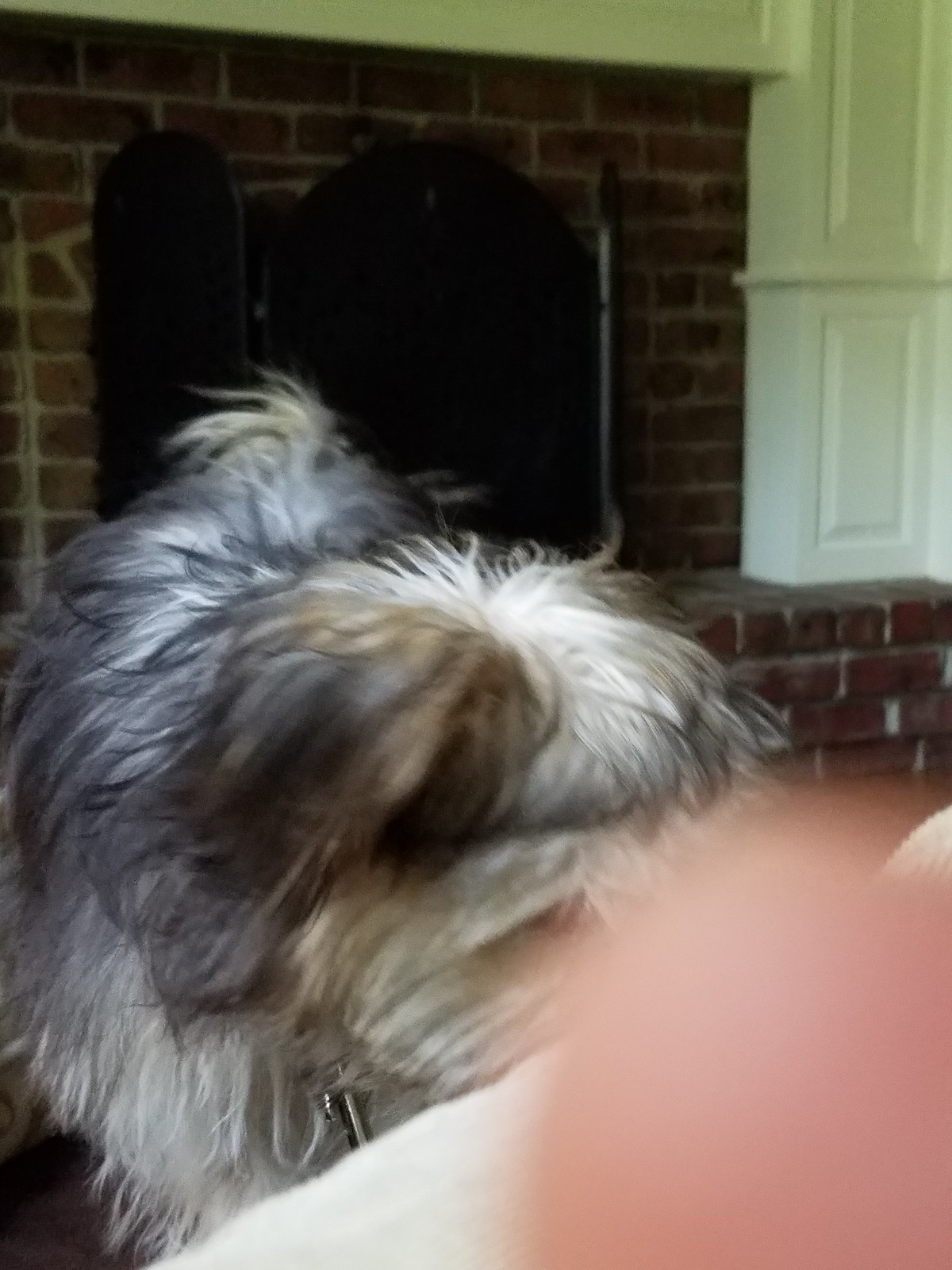In this somewhat blurry photo, a small, shaggy dog of a hairy breed is the focal point. The adorable canine has long fur in shades of white, tan, and possibly a hint of gray, with tufts so abundant that they obscure its eyes. Positioned in the lower right-hand corner of the image is a skin-colored blur, which might be a finger or knee, indicating a very close perspective. The dog stands near a chimney, partly concealed by a black structure in front of it. Despite the blur, the dog's fluffy tail is discernible in the background, contributing to the overall charming disarray of the scene.